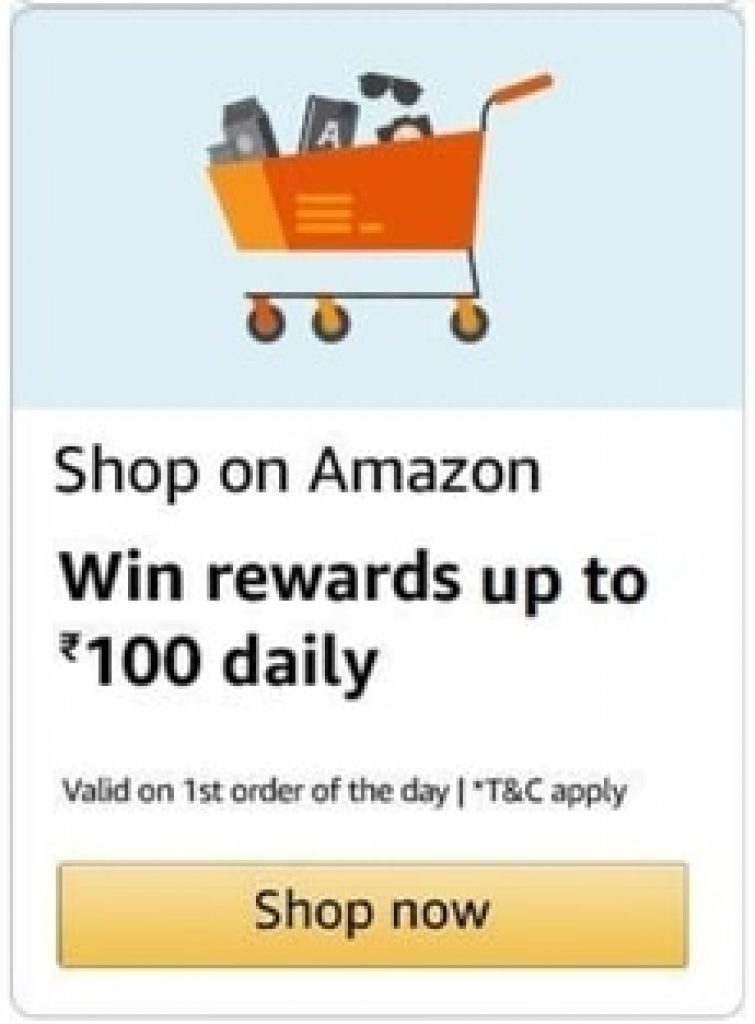This is a highly magnified screenshot of an Amazon promotional window, originally designed to be a small rectangle but inexplicably scaled up by approximately 400-600%. The image displays a gray-bordered, rectangular interface. The upper third of the window features a light blue background, partially overlaid by an orange shopping cart icon filled with various items including a carton of milk, sunglasses, and several other small products. Below the cart, the text reads "Shop on Amazon." 

Further down, in bold, is the message: "Win rewards up to 100 R" (likely rubies) followed by a note that specifies, "Valid on first order of the day. TNC apply," indicating terms and conditions apply. At the bottom of the window is a prominent yellow "Shop Now" button.

The image quality suffers greatly due to the excessive magnification, resulting in significant graininess, noise, and pixelation, which distorts the text and overall clarity. Details such as the three wheels of the shopping cart, its black-barred orange handle, and its lighter orange front in contrast to its darker side panels are discernible despite the poor image quality.